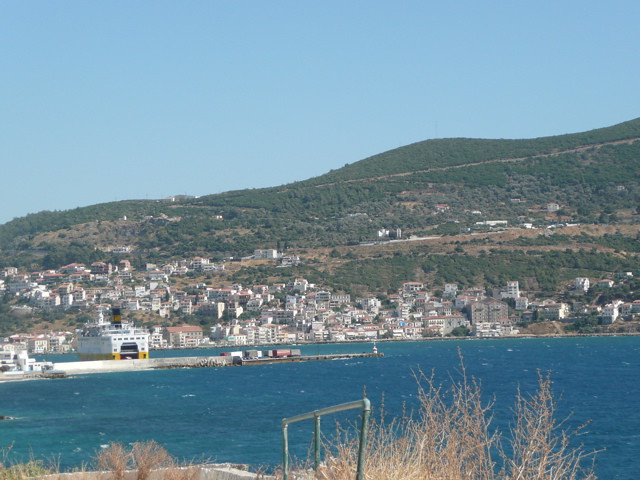This image showcases a picturesque waterfront city nestled against a hillside, viewed from the opposite shore. In the foreground, a metal railing lines the edge, framing the vibrant blue water that stretches across the scene. Near the shore, a large cruise ship is docked, its presence dwarfed by the sprawling expanse of the city and its surroundings. The middle of the water features a pier-like structure, adding depth to the composition. The city's cluster of white buildings, many topped with red or orange roofs, sprawls across the hillside, indicating a densely populated area. Trails and possibly drivable roads snake up through the lush, wooded hills and mountains that rise behind the city, providing a stark natural backdrop to the urban landscape.